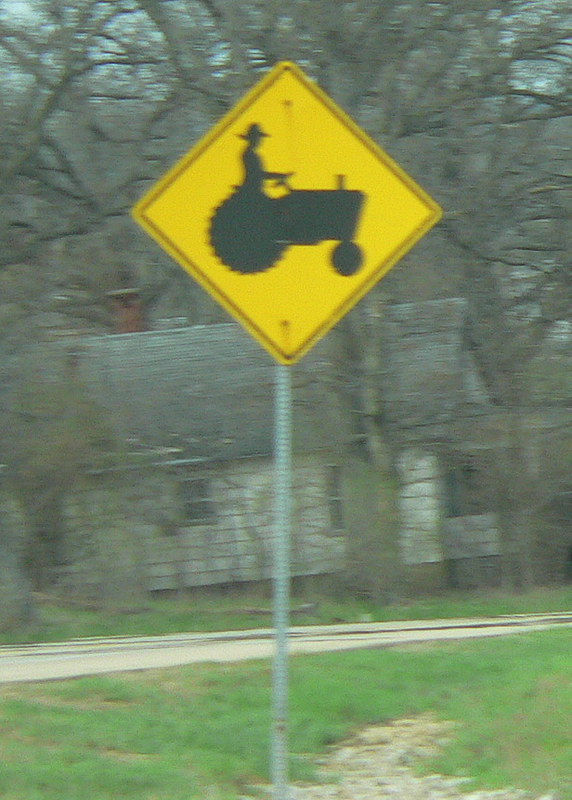In this low-resolution image, the focal point is a triangular, diamond-shaped, yellow warning sign situated in a grassy or dirt lot. The sign prominently features a black silhouette of a man wearing a farmer's hat and driving a tractor, indicating it's likely a caution sign for agricultural activity. The base of the sign is not visible, but the four-pointed shape is clear. The background of the image is slightly blurry, with a road cutting across the frame horizontally. Beyond the road, there's a modest, one-story house surrounded by sparse trees that appear to have shed their leaves, suggesting the photo was taken in the fall or winter. The overall scene exudes a rural atmosphere, reinforced by the presence of the sign, the isolated house, and the barren trees.